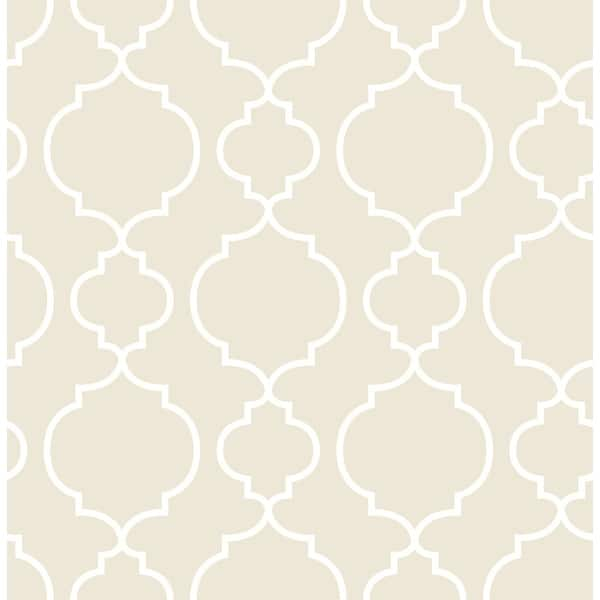The image depicts a detailed wallpaper design with a cream-colored background. The primary pattern consists of a series of vase-like, globe-shaped structures that are outlined in white. These shapes have rounded edges with pointed tips at both the top and bottom, forming an interconnected pattern. Each row alternates in size, with the larger shapes interspersed with smaller ones, creating a visual rhythm across the wallpaper. The rows of this intricate pattern stretch vertically, with five in total, although the shapes on the far left and right edges appear partially cut off. The repeating design forms an overarching pattern that resembles a flowing riverway. The simplicity of the cream and white color palette enhances the elegance and subtlety of the design.